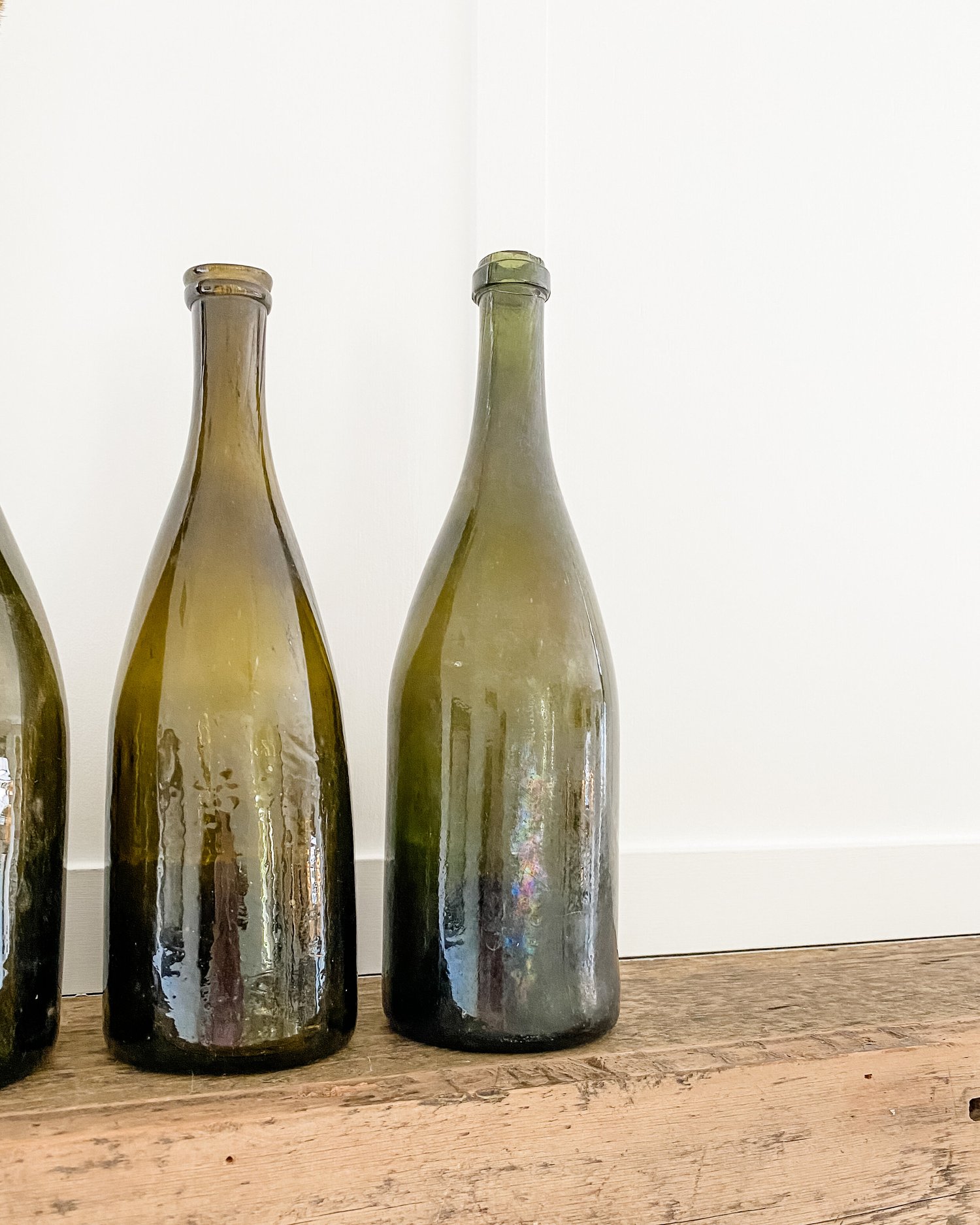In this color photograph taken in portrait orientation, we see three tall, empty green glass bottles positioned on a weathered wooden platform against a white wall. The center bottle, an olive green and the largest of the three, stands open with no cap. To its right, a darker green bottle is sealed with a visible cap. On the far left, a third bottle is partially visible, slightly amber in color. The aged wooden platform, light beige in color, adds texture to the composition. Light reflections and the faint outline of opposite furniture and walls can be seen on the smooth surfaces of the bottles, which lack labels and hint at resembling wine bottles. The photo, taken at a slight angle, captures a sense of realistic representation and simplicity.